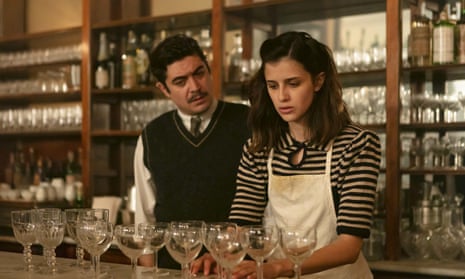The photograph captures an indoor bar setting where a man and a woman are positioned behind a counter adorned with numerous goblet-like glasses, which are arranged from the woman's front to the left edge of the image. The man, appearing slightly behind and to the left of the woman, has short black hair and a mustache, and is dressed in a dark sweater vest over a white shirt with a tie. His head is cocked slightly to the right, giving the impression that he is observing the woman closely. The woman, standing closer to the camera, has shoulder-length brown hair and is wearing a black and white striped shirt with sleeves extending to her elbows, topped with a white apron. She appears to be looking down and slightly to the left with a concerned or confused expression on her face. Her hands rest on the tan and white countertop. Behind them, the bar shelves are lined with glassware and various bottles, adding to the ambiance of the bar environment. The overall scene suggests a dynamic where the woman might be uncertain or troubled, while the man seems to be either watching her actions intently or possibly reprimanding her.